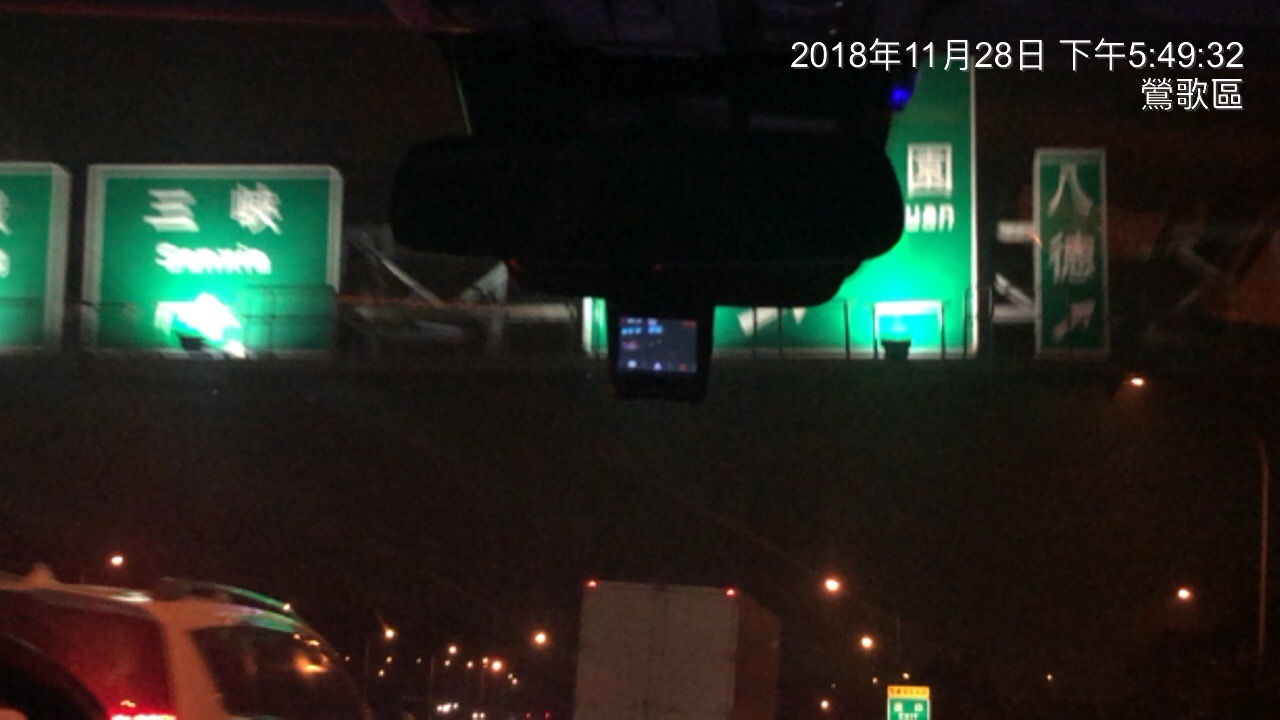A nighttime scene captures a somewhat incomplete and blurry image of a highway, cluttered with multiple overhead green road signs. The pitch-black sky forms the backdrop for these signs, which are framed with white edges. On the left, there appears to be a partial sign, adjacent to another green sign that contains indistinct white text in the center. A metal steel pole traverses the frame horizontally, intruding into the visibility of a small segment of an additional sign and what seems to be an information screen.

Further right, another large green sign is discernible but only a small portion is visible; the central part of this sign is missing due to the incomplete view. Next to this is a section of another metal pole and a smaller rectangular green sign featuring white symbols. Below this, the black sky is prominent, while in the lower left corner, the top of a car and its lights are faintly visible.

In the distance, a box truck drives along the road, accompanied by another smaller green roadside sign that is partially visible. The dim lighting and motion blur add to the scene's nocturnal ambiance, capturing the hustle of nighttime highway traffic.